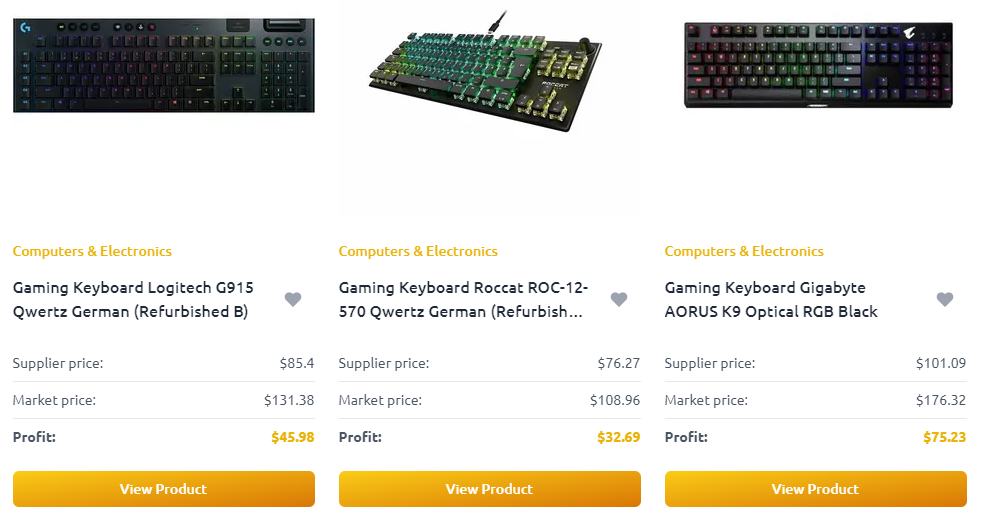The photograph captures an online sales platform, distinct from Amazon in its interface layout. Featured prominently are three different gaming keyboards, each with its own unique attributes and pricing details.

1. **Gaming Keyboard Logitech G915 Quartz**:
   - **Category**: Computers and Electronics
   - **Condition**: German Refurbished
   - **Supplier Price**: $85.40
   - **Market Price**: $131.38
   - **Profit Margin**: $45.98
   - **Description**: A sleek gaming keyboard under the Logitech brand, positioned for quick access through a "View Product" bar.
   
2. **Gaming Keyboard Roccat ROC 12570 Quartz**:
   - **Category**: Computers and Electronics
   - **Condition**: German Refurbished
   - **Supplier Price**: $76.27
   - **Market Price**: $108.96
   - **Profit Margin**: $32.69
   - **Description**: This keyboard features visually striking, elevated key design with internal lighting, enhancing the gaming experience.

3. **Gaming Keyboard Gigabyte Aorus K9 Optical RGB Black**:
   - **Category**: Computers and Electronics
   - **Condition**: New (presumably)
   - **Supplier Price**: $101.09
   - **Market Price**: $176.32
   - **Profit Margin**: $75.23
   - **Description**: An advanced gaming keyboard with dynamic RGB lighting, providing a visually immersive and high-tech appeal. 

Each keyboard, appealing to gaming enthusiasts, is highlighted with its respective profitability and condition, aimed at helping shoppers make informed decisions.